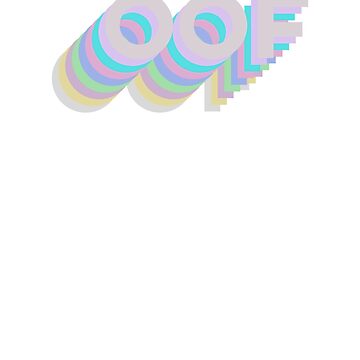The image features a pixelated, computer-generated logo positioned towards the top of an all-white background. The logo reads "OOF" in capital letters and appears to have a 3D effect as if it's coming off the screen. Each letter of "OOF" is shadowed by a pixelated, rainbow spectrum that includes colors such as white, light blue, pink, purple, light green, darker purple, yellow, turquoise, and orange. The letters are upright and centered horizontally, creating a simplistic yet vibrant visual against the otherwise blank backdrop. The overall style suggests that it could be a piece of clipart or an image from a stock photo website.